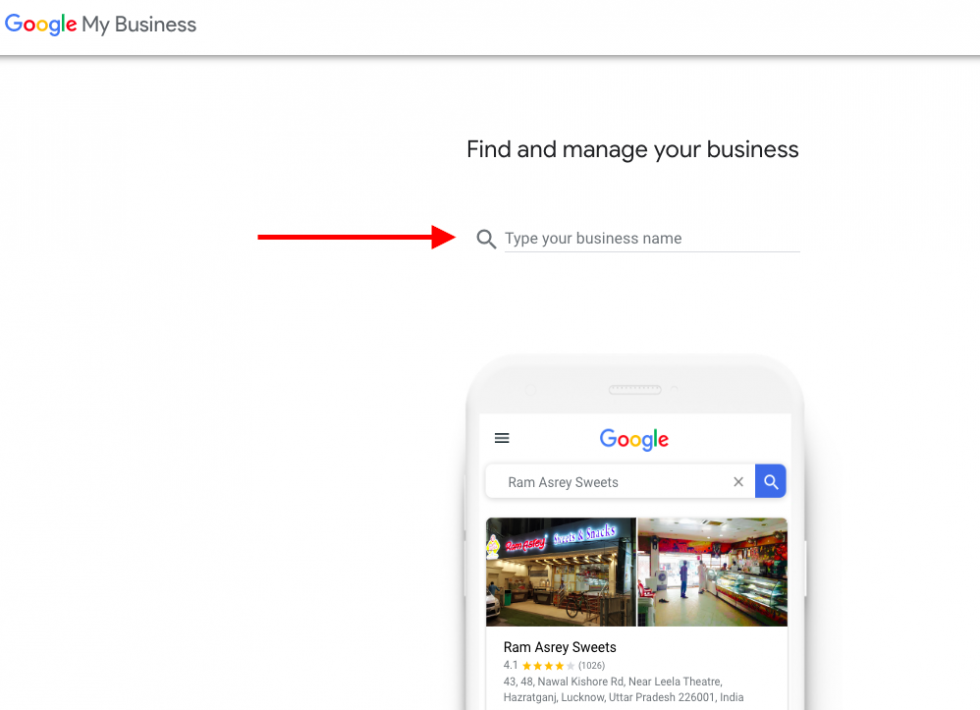The image is related to Google My Business and features a clean, white background with no borders. In the top left corner, the text "Google My Business" is displayed. A gray line spans the width of the image just below the title, followed by the text "Find and manage your business" in a clear, readable font.

A prominent red arrow points towards a search bar, which contains a magnifying glass symbol and the instruction "Type your business name" inside the bar. Below the search bar, the top portion of a smartphone, depicted in a whitish-light gray color, shows the familiar Google logo in colorful letters. The search bar on the smartphone displays the text "Ram Asri Sweets."

Beneath the search bar, two images showcase the sweet shop "Ram Asri Sweets." The left image shows the exterior of the store, identifiable by signage that mentions sweets and snacks. The right image provides an interior view, where a few people are seen standing near a large display case filled with various food items.

At the bottom of the image, the text "Ram Asri Sweets" is displayed along with a rating of 4.1 stars. The address "4348 Nawal Kishore Road near Lila Theater, Hazragad, Lucknow, Uttar Pradesh, India" is provided, clarifying that this sweet shop is located in India.